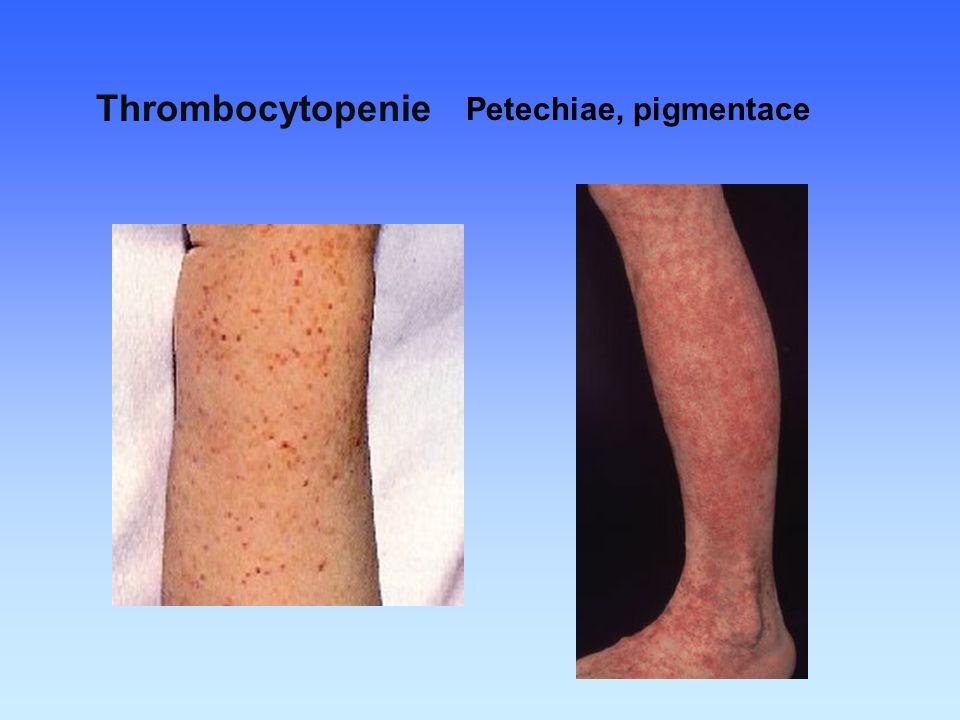The image depicts a medical representation of thrombocytopenia petechiae pigmentosa, overlaying an ombre blue background transitioning from bright blue at the top to light blue at the bottom. The visuals include two photographs of extremities displaying symptoms: the left photo appears to be of a forearm, showcasing red indented dots characteristic of the condition, while the right photo shows a leg from the knee to the foot, with blotchy red skin. Both pictures have captions above them, detailing the disorder. The overall setting appears clinical, likely indoors, emphasizing the skin abnormalities for educational or diagnostic purposes.